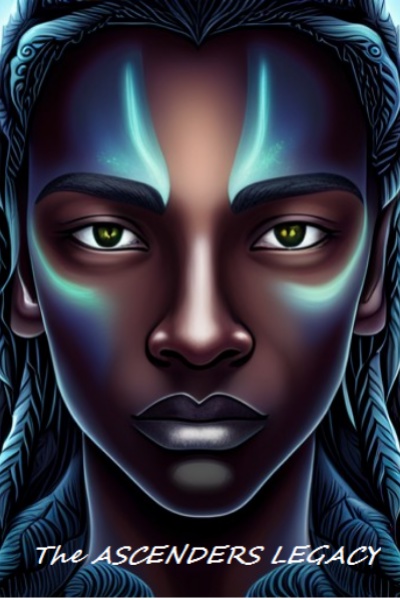This is a vertically-oriented, digital illustration, likely a cover for a publication such as a book or magazine. The image features a portrait of an African American youth, possibly a teenage girl. She has striking greenish-brown eyes and an intense, serious expression. Her hair is intricately styled in braids or dreadlocks, adorned with fanciful, floral-like curlicues. Her dark brown skin is accented with symmetrical, metallic blue face paint that gives off a shiny, almost robotic appearance. This paint extends around her eyes, across her forehead, and along her cheekbones, creating a futuristic, sci-fi look. Her lips have a silvery, greyish-blue hue. At the bottom of the image, in white font, the text reads "THE ASCENDER'S LEGACY," with "the" in lowercase and "ASCENDER'S LEGACY" in uppercase.